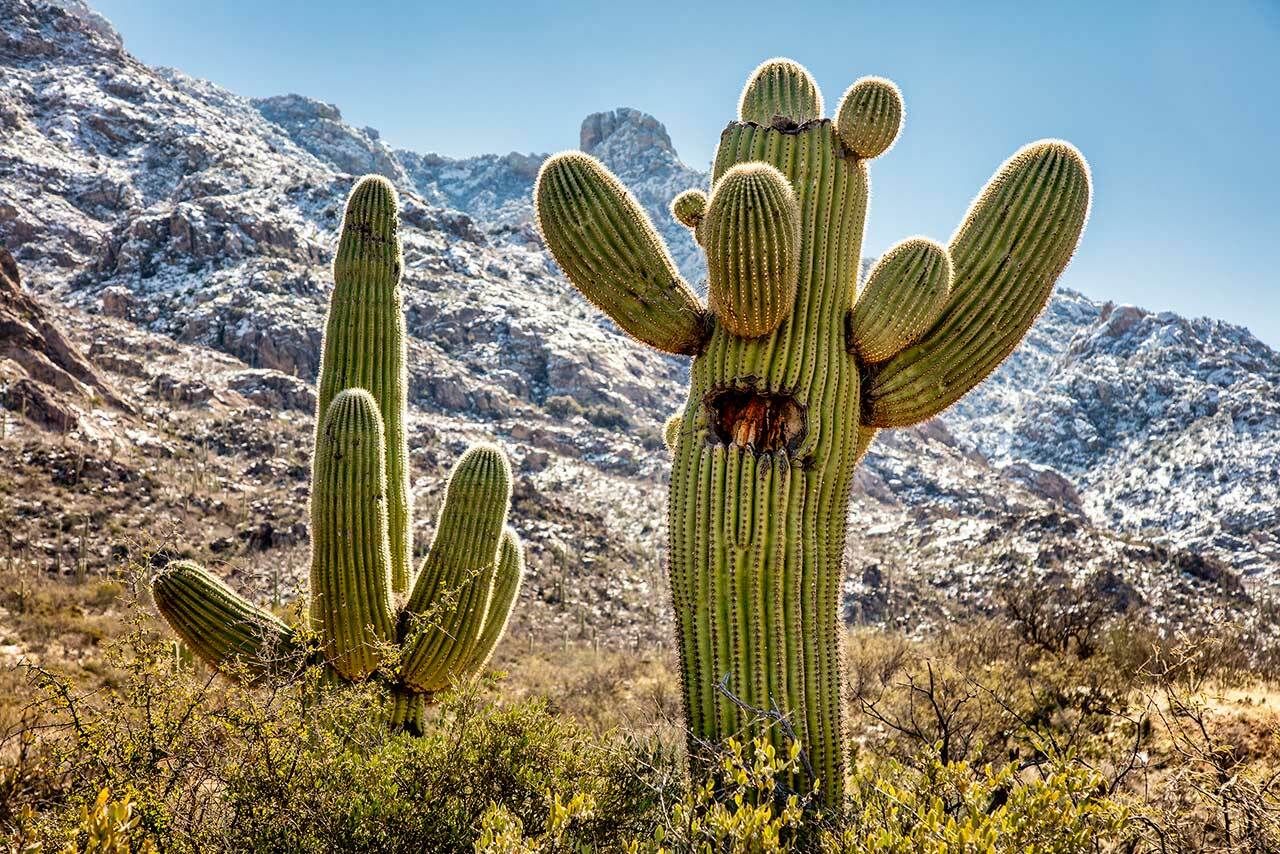In this photograph of a desert scene, the foreground features arid soil with scattered desert bushes and two prominent cacti. The cactus on the left is tall and straight, while the one on the right is a distinctive saguaro cactus with numerous arms sprouting from its sides and top. The saguaro cactus has a hollowed-out, round section in the middle, possibly indicating an animal burrow or some damage, as it appears slightly charred or rotted around the edges. The cacti's green surfaces are ridged with spines. In the background, a significant rock outcropping or hillside is visible, displaying shades of white, brown, and gray, which resemble snow or ash. Above, the sky is a light blue, suggesting a sunny, dry day with the sun harshly beating down on the landscape. The entire scene exudes the harsh, arid beauty of the desert, with the majestic cacti standing resilient against the stark, rugged backdrop.